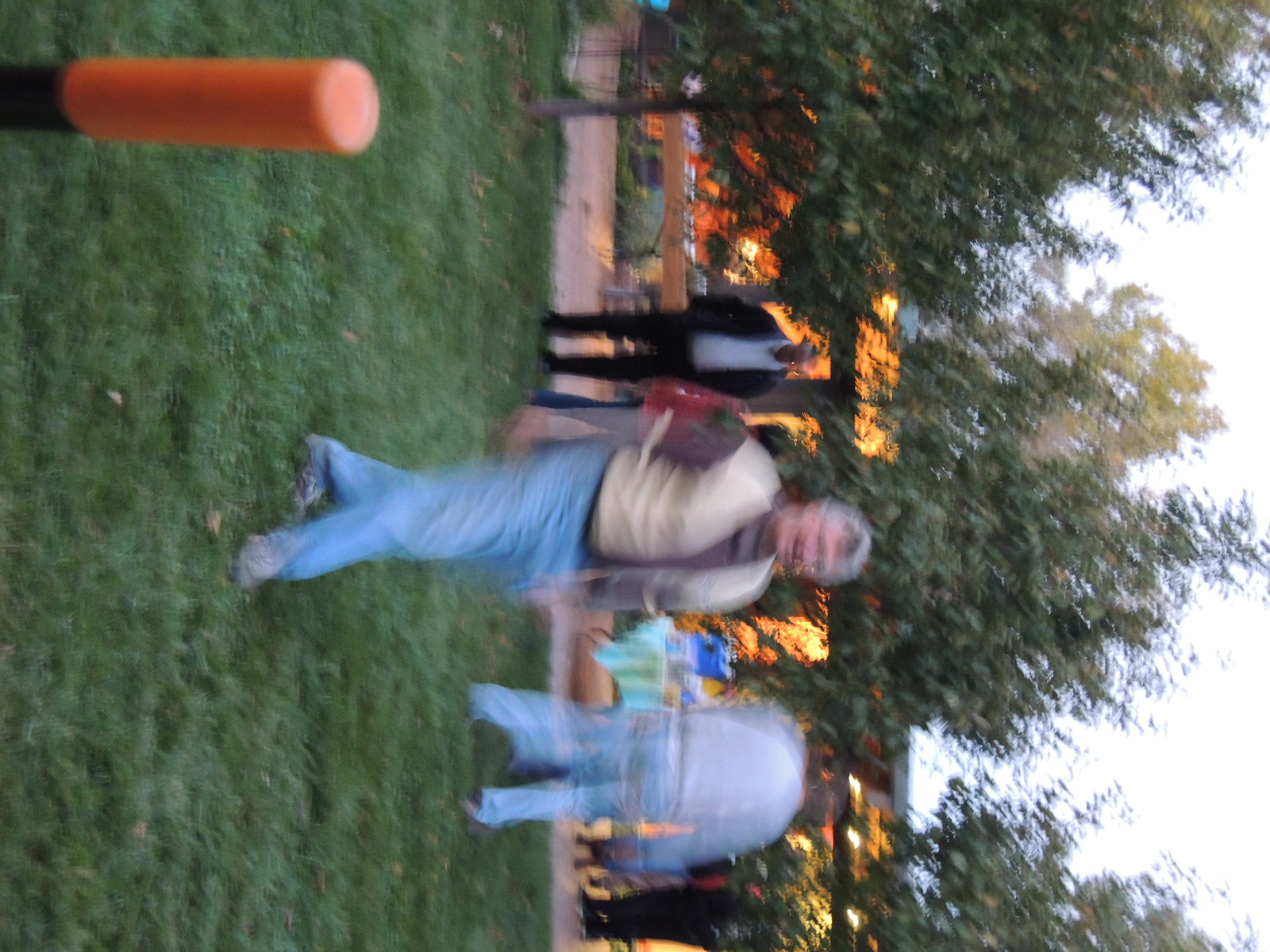The image, although blurred and turned sideways, captures an outdoor scene with rich green grass appearing prominently on the left. At the center of the photo stands an older Caucasian man with salt-and-pepper hair, possibly sporting a mustache and glasses. He is dressed in light blue jeans, gray sneakers, and a white vest over a combination of gray and brown shirts. Flanking him are two other men: one to his right in black pants, a black jacket, and a white shirt, and another to his left clad in blue jeans and a sweatshirt. Notably, an orange cylindrical pylon appears towards the upper right corner of the image due to its orientation. The backdrop features a row of trees with lush green leaves, hinting at spring or summer. Amongst this foliage, a brightly lit structure, perhaps an outdoor pavilion or storefront, can be spotted, accompanied by blurred tables resembling market stalls. The sky above appears washed out from sunlight, contributing to the light and exposure challenges in the photo.